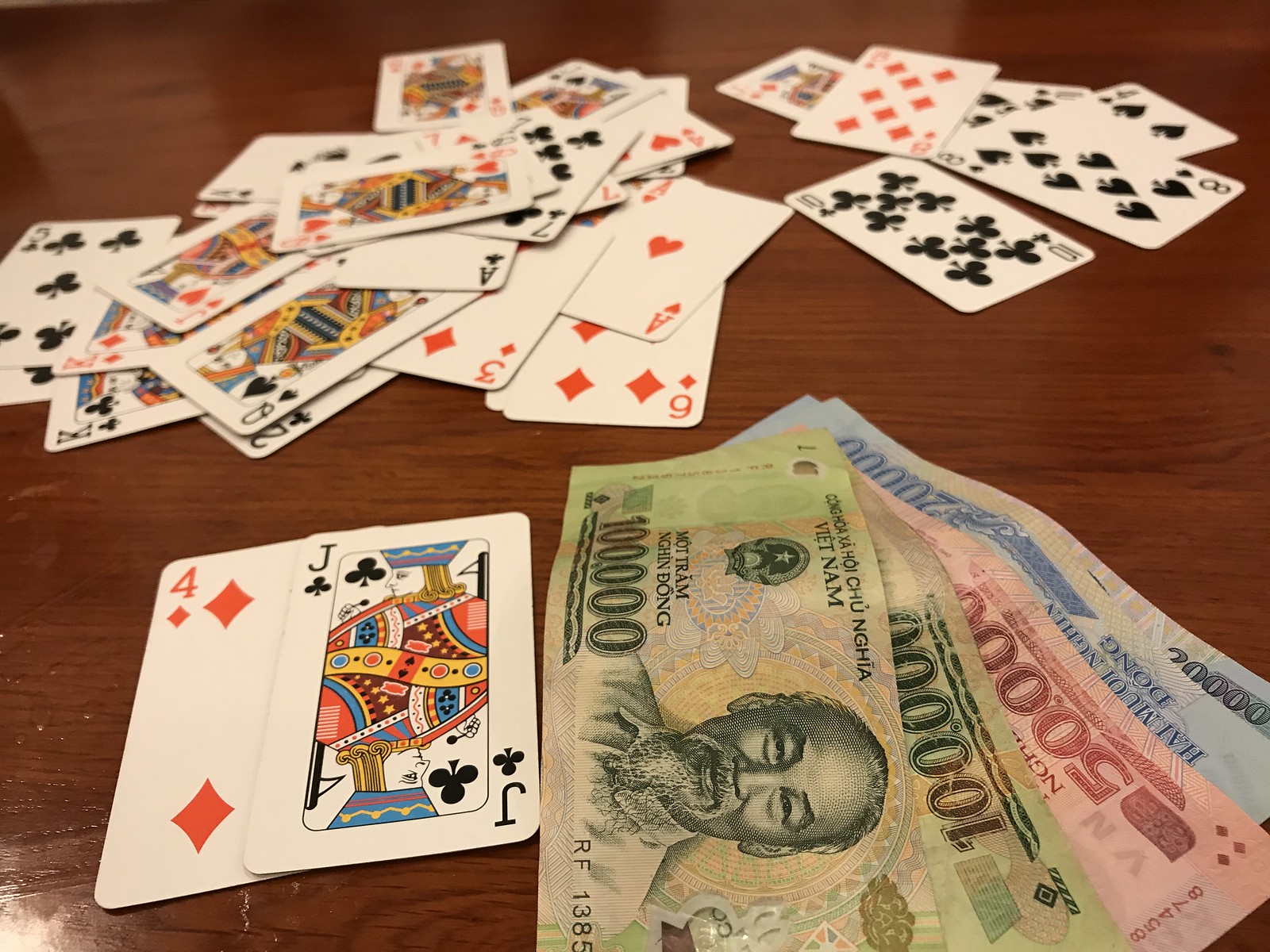The image is a realistic, horizontally framed photograph capturing a chaotic tabletop scene. The background showcases a richly textured wooden table, featuring varying shades of dark to medium brown with prominent dark brown grain patterns. Scattered across the table are numerous playing cards, all face-up with white backgrounds. 

In the bottom left corner, a four of diamonds card with bold red diamond icons is visible. Adjacent to it, towards the right, is a jack of clubs, intricately outlined in black and filled in with vibrant hues of yellow, red, and blue. 

Further into the scene, a sizeable disorganized pile of around 10 to 20 cards lies, showing a mix of red and black suits including cards like 10s, 8s, queens, and jacks. Another smaller cluster of five or six cards is situated to the right of this central pile.

In the bottom right corner of the image, several paper bills are laid out. There are two green bills, one red bill, and two blue bills. The topmost green bill, prominently featuring black text that reads "10,000" and marking it from Vietnam, includes a depiction of an elderly Asian man dressed in a white shirt. The bottom part of this bill, tilted with its bottom side facing leftwards, bears the black text "RF-1385" near the center.